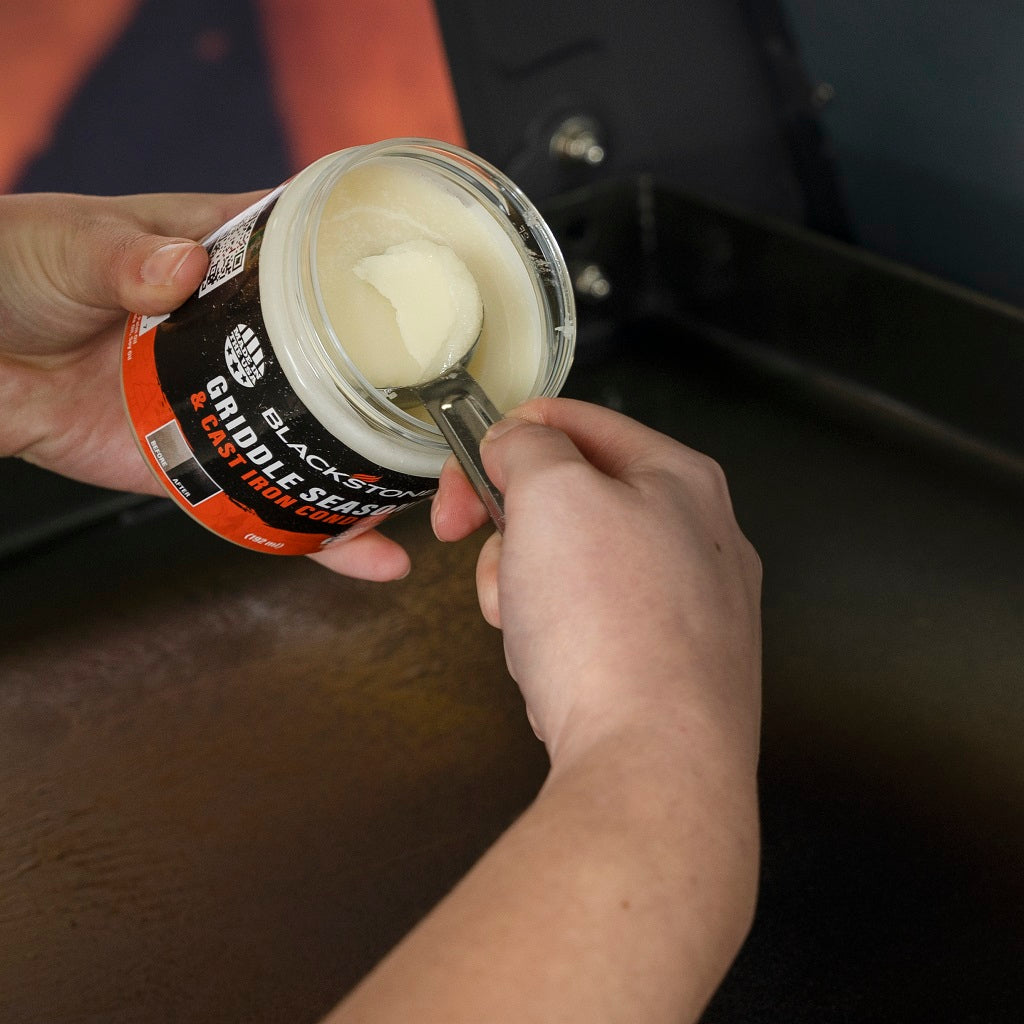The detailed image depicts a white individual’s hands, with a focus on their right and left hands and forearms. One hand grasps a container while the other uses a silver metal scoop to extract a substantial amount of an off-white, thick, creamy substance from a circular glass jar. The jar features a label with the brand name "Blackstone" in white text against a black background, followed by the words "griddle seasoning and cast iron conditioner" in orange text. The action suggests the person is preparing to season a cooking surface, likely a black flat-top griddle, as would be found in a commercial kitchen. The background seems to be a flat table surface, although it's unclear if the photo was taken indoors or outdoors. The scene embodies a culinary task, with the individual poised to rub the scooped-out substance on the griddle, emphasizing the preparation and maintenance of cooking equipment.